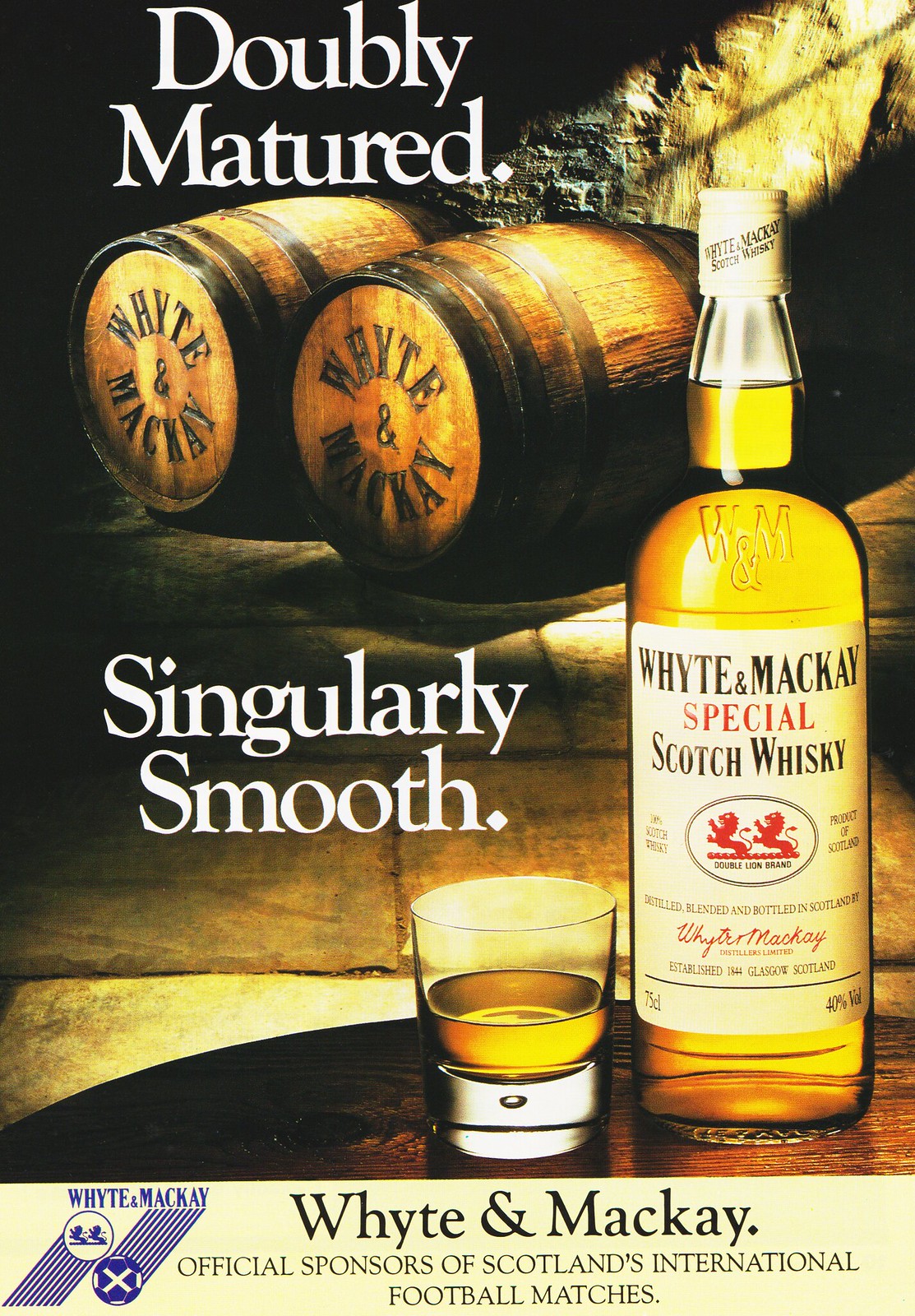This advertisement for Whyte and Mackay Special Scotch Whiskey predominantly features a golden hued theme. At the very top in white letters, the tagline "Doubly Matured" is displayed. Just below, two whiskey barrels are prominently shown, labeled "White and Mackay." Beneath the barrels, the phrase "Singularly Smooth" is highlighted in white. 

Centrally positioned at the bottom of the image is a glass of the featured Scotch, with the actual tall bottle of golden Scotch placed to the right. The bottle, etched with "W&M" just under its nozzle, bears a label with a white background. The label reads "Whyte and Mackay" in black, "Special" in red, and "Scotch Whiskey" in black underneath. An emblem featuring two red lions encased in a circle is prominent, marked "Double Lion Brand." Additionally, it details a strength of 40% volume and confirms its origin with "Product of Scotland" to the right of the emblem.

Towards the bottom on a light yellow background, in black letters, it is declared that Whyte and Mackay are the "Official Sponsors of Scotland's International Football Matches." The entire image is bathed in tones of yellow, gold, and brown, reinforcing the premium and refined nature of the Scotch Whiskey.